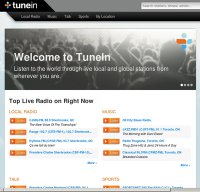This image depicts the homepage of the TuneIn website. In the top left corner, the website's name, "TuneIn," is prominently displayed in white text against a black background. On the top right, there is a search bar alongside several tabs, though the specifics of these tabs are not visible. 

A warm welcome message reads, "Welcome to TuneIn. Listen to the world through local and global stations here and wherever you are," though the text appears slightly unclear. Behind this message, a lively scene featuring people dancing with their hands raised fills the background, shaded in grey tones.

The TuneIn logo, featuring a mix of light blue, blue, and orange colors, is also visible. At the bottom of the page, a section titled "Top Live Radio On Right Now" is displayed, followed by categories such as local radio, podcasts, sports, music, and talk. These category titles are presented in blue text, but the specific details underneath each category are not clearly distinguishable.